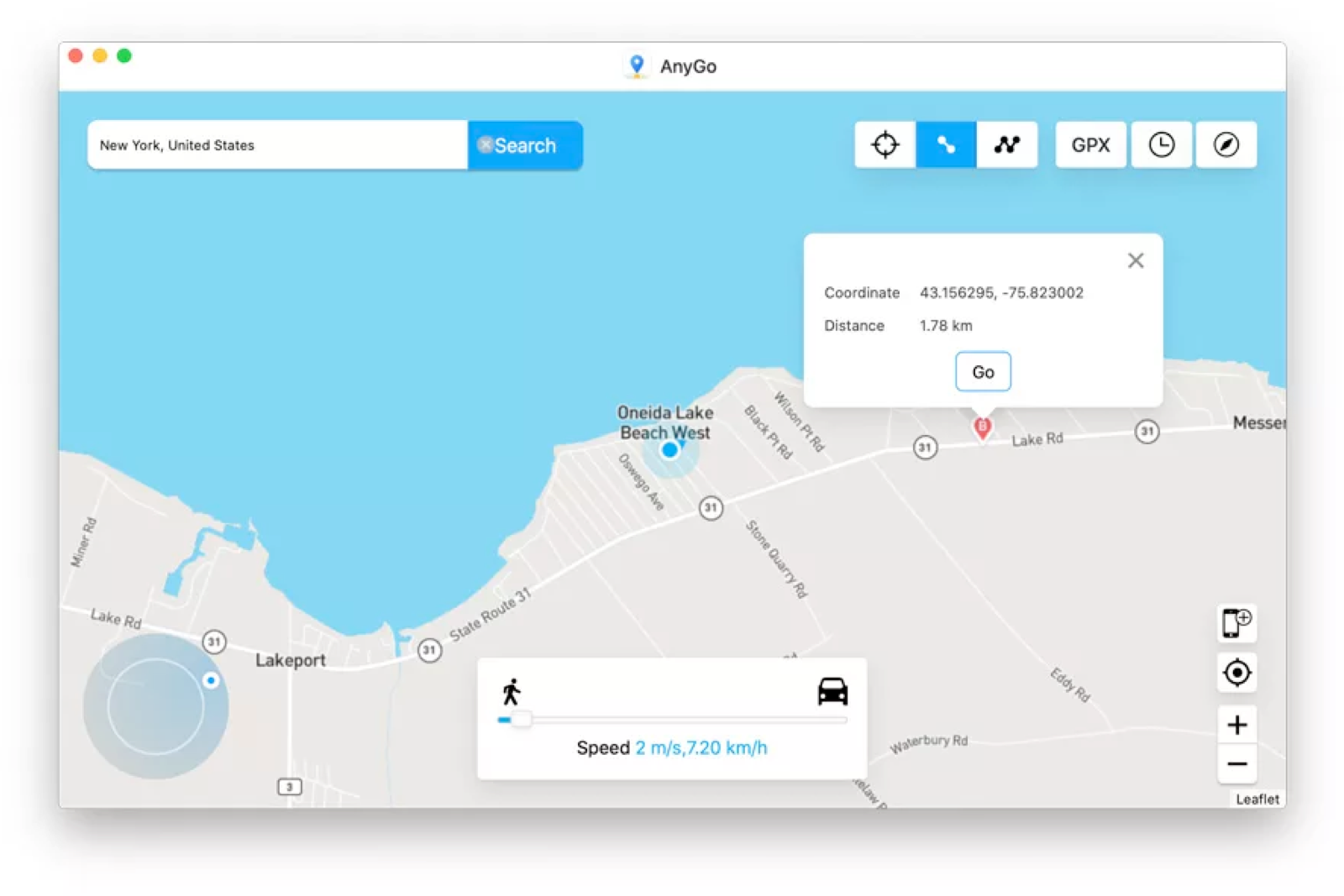The image depicts a detailed navigational map interface. The background is primarily blue water, indicating a lake, with several colorful markers and annotations.

In the very top left corner, there's a cluster of symbols: a red dot, a yellow dot, a green dot, and a white bar. The white bar is labeled "New York, United States." Adjacent to these icons is a blue pin and an annotation labeled "any cone."

Central to the map is a white bar with the text "New York, United States" and a blue button labeled "search." There is also a white square featuring a crosshair in the center, accentuated by blue and black elements. Nearby, a white "x" indicates a GPX file format.

Below are various symbols: a circle, a square with a colon, and a compass icon. Adjacent to these, a blue square displays the text "coordinate," indicating the map's current coordinates: 38.156295, -75.823002, with a noted distance of 1.78 kilometers.

A blue border and cone highlight the area, marked as "Oneida Lake, Beach West." There's a blue dot pinpointing specific locations along "Lake Road" and "Lake Park," intersecting at "State Route 31."

At the bottom, the map shows a person walking towards a car with their speed displayed as 2 meters per second (7.20 kilometers per hour). This is annotated as a pin at "Oneida Lake, Beach West." The map further shows routes, including "Lake Road" and "State Route 31."

Additional map icons include a smartphone symbol, a pin, and a plus and minus sign for zooming. The bottom portion of the map interface displays a gray bar, completing the layout.